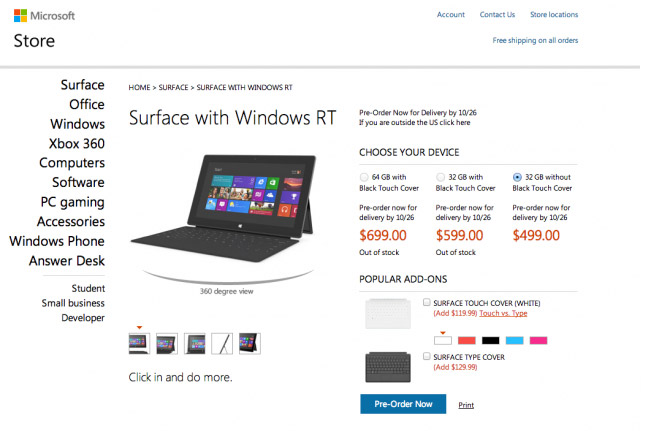This is a meticulously detailed screenshot from the Microsoft Store's webpage. In the top left corner, the heading "Microsoft Store" is visible, while the top right corner features links for "Account," "Contact Us," "Store Locations," and "Free Shipping on All Orders." A vertical menu on the left lists various Microsoft product categories such as Surface, Office, Windows, Xbox 360, Computers, Software, PC Gaming, Accessories, Windows Phone, Answer Desk, Student, Small Business, and Developer.

Centered in the image is a high-resolution picture of a sleek black Surface laptop, propped up with an attached black keyboard. Above the laptop image, "Surface with Windows RT" is prominently displayed, with a curved underline leading to the text "360-degree view. Click in and do more."

To the right of the laptop image, a compelling call-to-action encourages users to "Pre-Order Now for Delivery by 10/26," along with an option for users outside the U.S. to click a provided link. Additionally, customers can choose their preferred device configuration:

1. 64 GB with Black Touch Cover: Pre-order for delivery by 10/26, priced at $699 (currently out of stock).
2. 32 GB with Black Touch Cover: Pre-order for delivery by 10/26, priced at $599 (currently out of stock).
3. 32 GB without Black Touch Cover: Pre-order for delivery by 10/26, priced at $499 (marked as selected).

Under the device options, the website invites users to "Pop your add-ons," listing accessories like the Surface Touch Cover in white for an additional $119.99 and a comparison between Touch vs. Type with the Surface Type Cover for an added $129.99. Users are urged to pre-order and to print the details for reference.